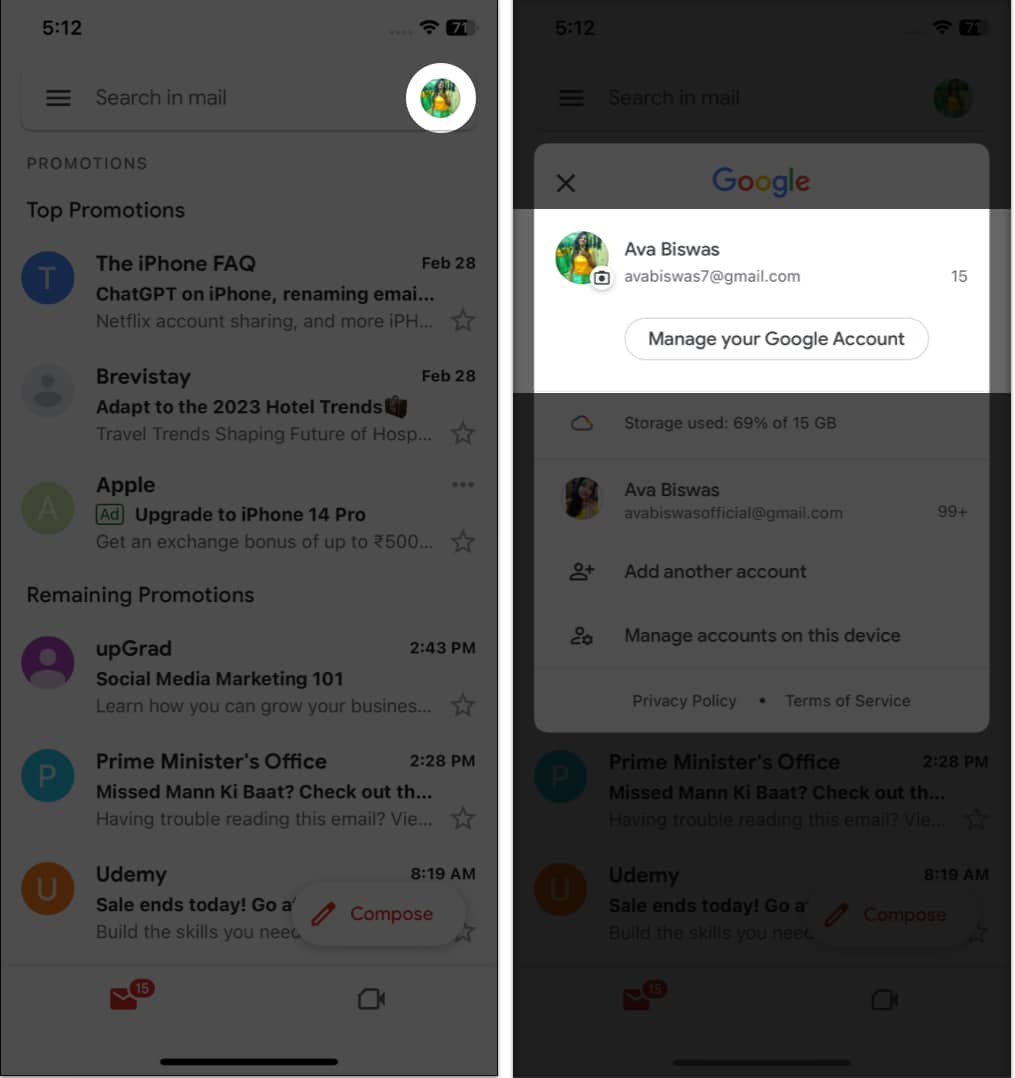The image depicts the screens of a cell phone, both featuring a gray overlay that dims the underlying content. On the left screen, the time is displayed as 5:12, and status icons for cell signal, Wi-Fi, and battery life (71%) are visible at the top. The main visible content on this screen is a white circular profile picture of a woman with long dark hair, wearing a yellow shirt and green pants.

The right screen features additional details. At the top, there is a white horizontally-elongated rectangle containing the same profile picture. Adjacent to this image, a photo icon is situated in the bottom-right corner of the circle, and the name "Ava Biswas" is displayed prominently, along with the email "AvaBiswas7@gmail.com" in a lighter gray font. To the right of this information, the number 15 is visible in gray.

Below this section, there's a lengthy white button outlined in gray, reading "Manage your Google account" in black text. Adding to the complexity of the layer is a darker gray overlay towards the bottom, beneath which appears to be a partially obscured, white rectangle and more content resembling the left screen's structure, but in an even darker gray tone.